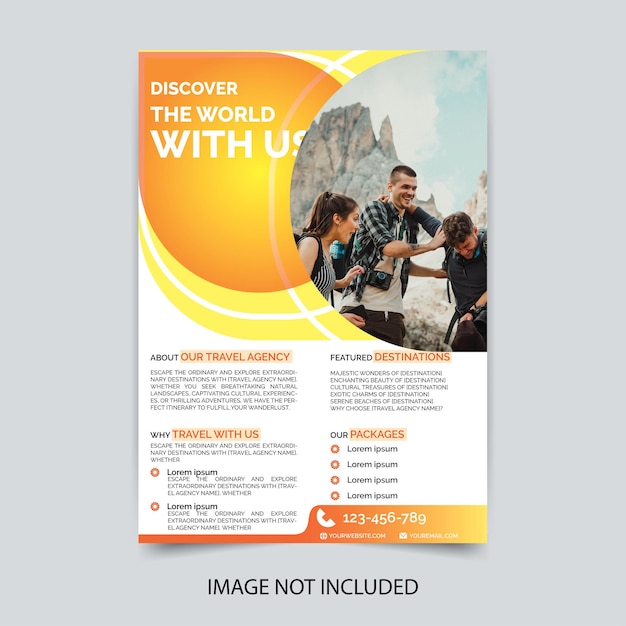The image is an advertisement template for a travel agency, featuring a vibrant background with orange and yellow orbs and white text that reads "Discover the world with us." The advertisement includes a prominent circular cutout containing a photograph of three friends—two young men and a woman—standing outdoors amidst mountainous terrain under a blue sky with scattered clouds. The friends appear joyful and ready for an adventure, dressed in hiking attire with backpacks; the woman on the left sports a white and black shirt with black straps from her bag showing, while the man in the middle is laughing and wears a blue and black plaid shirt. Various headings on the ad detail sections such as "Our Travel Agency," "Why Travel with Us," "Feature Destinations," and "Packages," each accompanied by placeholder text in English and Latin, indicating it's a template. At the bottom, there's a disclaimer that reads "Image not included," and in the lower right, an orange section displays a phone number. The ad employs a clean design with a harmonious color scheme incorporating black, white, red, orange, yellow, gray, green, and blue.